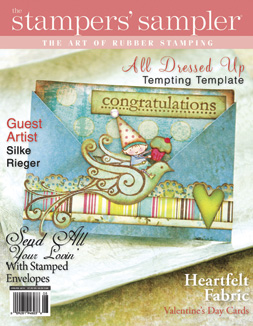This image is of a magazine cover for "The Stamper's Sampler." The title is prominently displayed in white text on a medium pink background, with the subtitle "The Art of Rubber Stamping" in white text against a light pink background just below it. Central to the cover is an illustration of a congratulatory card featuring a whimsical scene where a person in a party hat is riding a bird. The card is detailed with hearts and other decorative designs, indicating it is hand-stamped. Above this illustration, the text "All Dressed Up" is written in pink cursive, followed by "Tempting Template" in black text. On the left side, it mentions "Guest Artist Silky Ryder," showcasing the contributing creative talent. The lower right corner promotes "Heartfelt Fabric Valentine's Day Cards," and the lower left encourages readers to "Send All Your Creations in Stamped Envelopes." A barcode is situated at the bottom left of the cover. Overall, the cover highlights various artistic stamping techniques and projects, appealing to crafting enthusiasts.